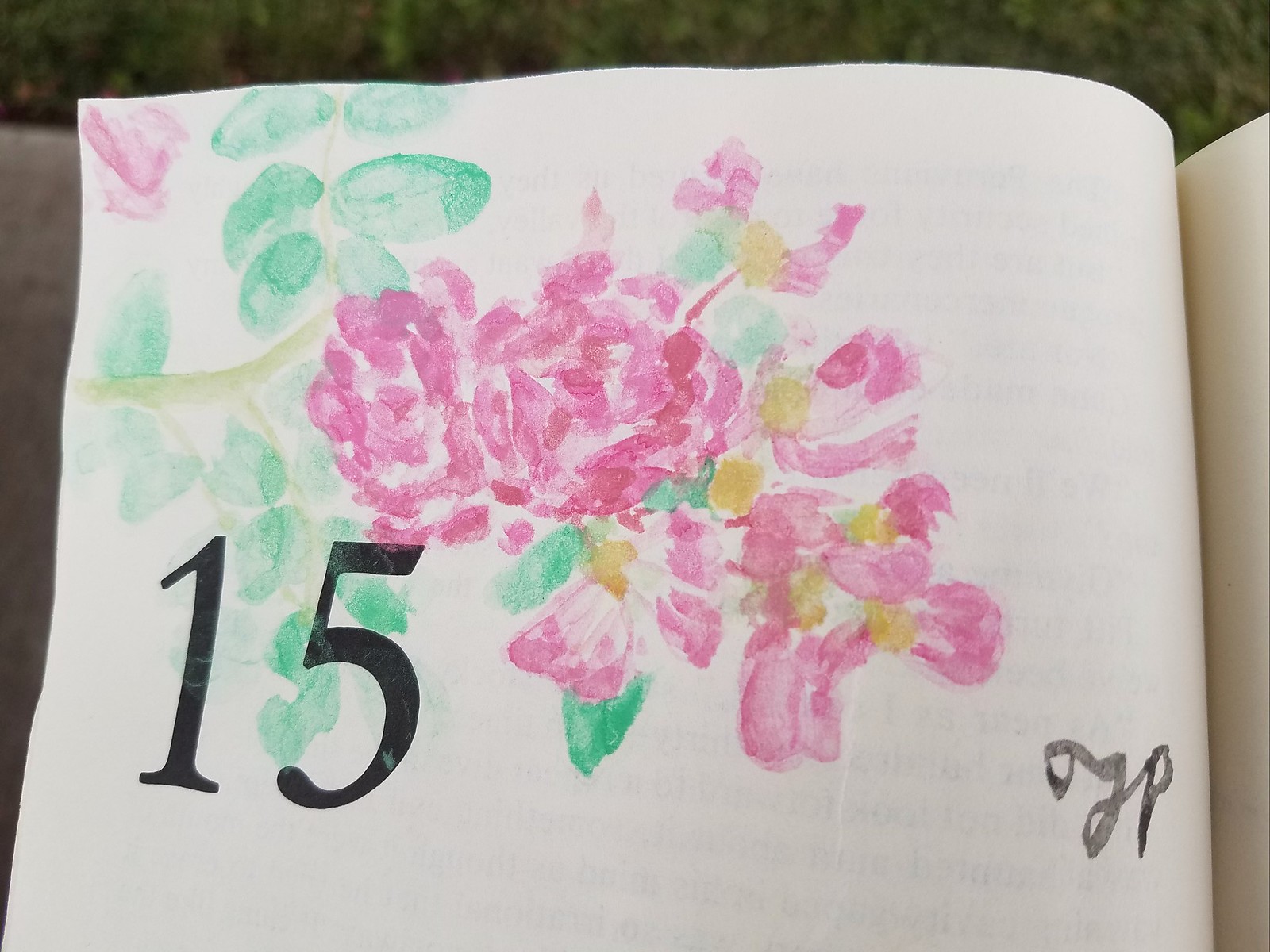This image depicts an open book, showcasing the top half of a page with a faint impression of black text visible through it. The main focus of the page is a delicate watercolor painting of a pink blossom with petals extending from a light green stem, accented by darker green leaves. The floral design features abstract petals with hints of pink and purple, interspersed with subtle gold inflections. To the left of the flower painting is a large, bold number "15," while towards the center-right of the page, in watercolor, are cursive initials "OGP" in lowercase, resembling a personal signature. The overall composition of the artwork appears pastel and light, with a natural, almost fingerprint-like application of green paint for the leaves.